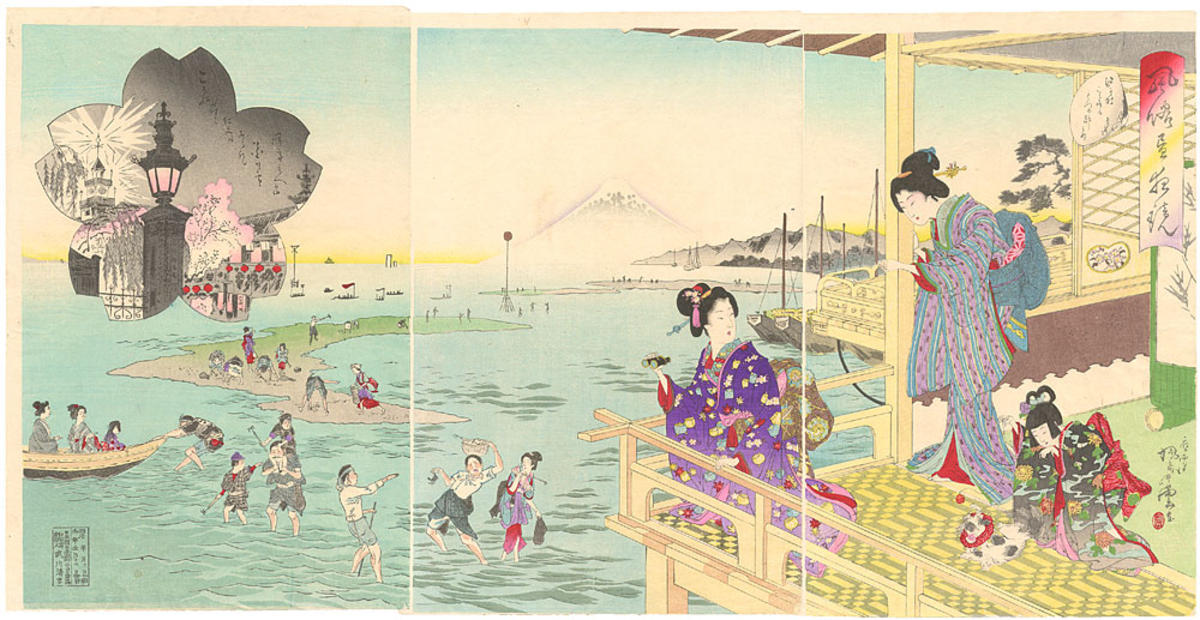This detailed and vibrant drawing captures a picturesque scene of a city and lake in East Asia, possibly Japan or China, framed by a blue and white sky. On the left side, a large, uniquely-shaped gray structure with a prominent white light perched on top towers over the scene. Below this structure, water stretches toward the foreground, where a small strip of land juts into view, occupied by several people enjoying playful activities. A boat, with one person pulling it ashore, nearly touches the bottom left corner as six more people frolic in the water behind it.

Dominating the right side of the drawing is the detailed depiction of an interior pavilion deck. A woman in a bright purple kimono kneels, facing toward the water, her head turned to engage with another woman standing behind her in a striped pink and blue kimono. At their feet, a young girl with short black hair, dressed in a black and red kimono, plays with a small dog. Colorful banners and flags hang from the pavilion's ceiling, adding to the festive atmosphere.

The image also features distant ships, one in the top left corner with an indistinct, gray, clover-like shape, and a mountainous or volcanic landscape rising in the middle background, enhancing the idyllic and leisurely scene. The overall color palette is notably pastel and faded, save for the vivid hues of the kimonos. The combination of intricate details, such as the geisha-like figures, the playful waterfront activities, and the serene natural elements, creates a captivating and richly descriptive tableau.